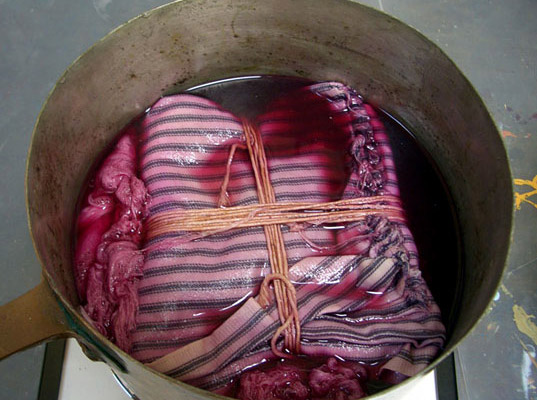This close-up photograph captures the intricate process of dyeing. At its center is a well-used silver bucket, marked with brown specks and scratches. Inside the bucket lies a shirt, bound by twine that crosses in the middle, tightly holding its shape. The shirt, primarily white with blue vertical stripes, is immersed in a reddish dye that envelops the fabric. To the left, the bucket's brown handle is visible. The setup rests on a white table with a black frame, set against a gray floor speckled with paint and dye stains, adding to the rustic and artistic atmosphere of the scene. The immersive colors and textures illustrate the detail and care involved in the dyeing process.